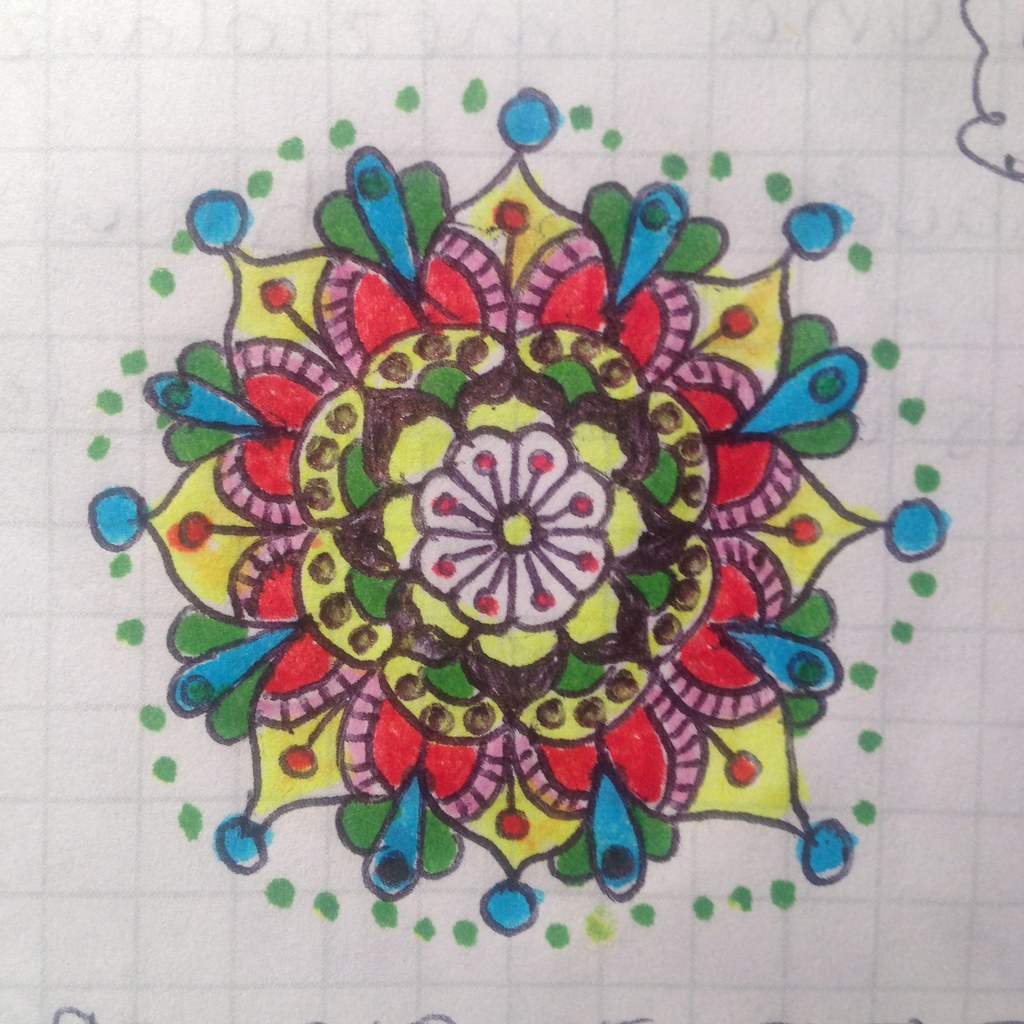The image displays a meticulously drawn flower on a sheet of graph paper, where the intersecting horizontal and vertical lines create a series of squares. The flower is composed of multiple layers of petals in a variety of colors, including pink, red, yellow, green, blue, and black. At its heart, the flower has a yellow center with eight surrounding petals, each adorned with red dots. Encircling this core is a set of eight yellow petals tipped with brown, followed by another layer of eight green petals. The bottom parts of these petals are green, whereas the tops are yellow with three brown dots each. Adjacent to this layer is a flower with eight red petals, each edged in pink stripes and featuring a central design resembling peacock feathers, with a blue teardrop flanked by two green teardrops. Beyond this lies yet another series of eight yellow petals, each marked with a red dot in the center and a blue dot at the tip. Encasing the entire floral structure is a ring of small green dots. The periphery of this artistic piece is accentuated with a black flower situated at the top right, rounding out the vibrant and detailed composition.